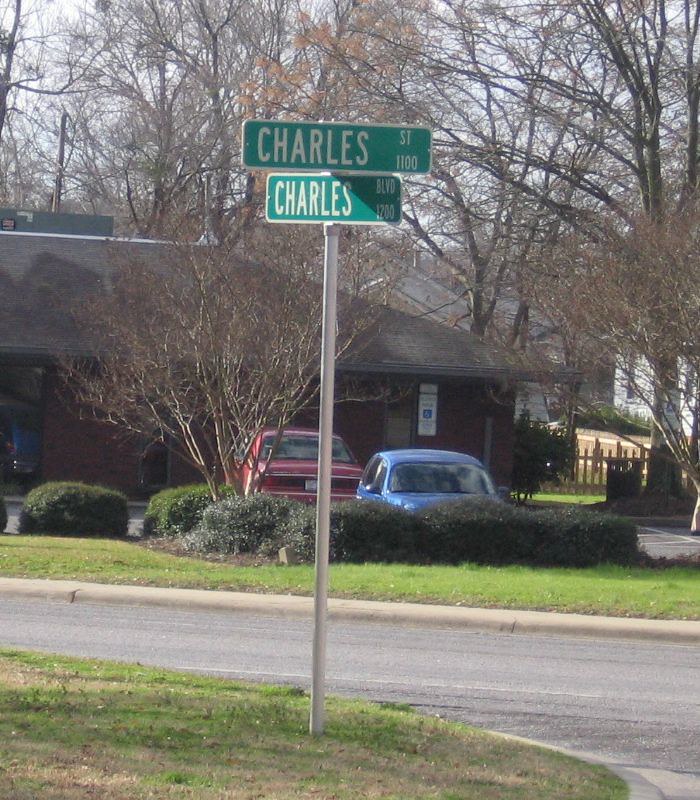In this color photograph taken outdoors, the focal point is a silver metal pole planted in the grass, supporting two green street signs with white, all-caps text. The top sign reads "Charles Street, 1100" and the one below it reads "Charles Boulevard, 1200." The backdrop includes a one-story brick building with a gray roof, likely a public building with handicapped parking. Beautiful green grass, hedge-type bushes, and a small tree enhance the foreground. Parked in front, there's a red car with a blue car behind it. The surrounding scene features additional trees, a brown fence, a couple of white houses, and a mix of green and bare patches of grass along the street corner where Charles Street intersects with Charles Boulevard.